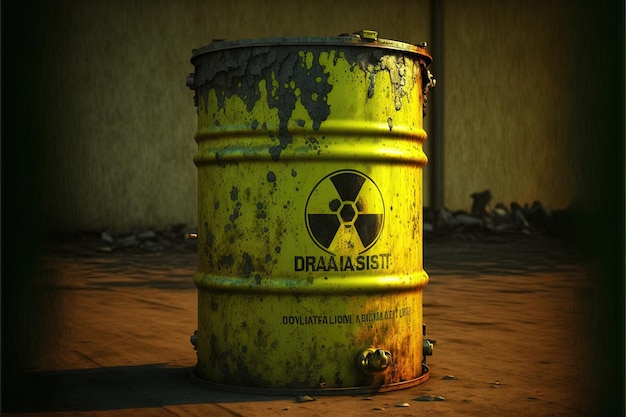This photograph, likely a digital creation or a video game screenshot, features a heavily corroded yellow 50-gallon drum of hazardous waste positioned in an indoor, dilapidated setting. The drum sits on a dark brown dirt floor strewn with various pieces of junk and rubble pressed against a dimly lit, streaked light gray wall in the background. A gray pipe extends upward along the wall, adding to the atmosphere of neglect. The yellow drum, marked by rust and dark brown ridges at both the top and bottom, prominently displays a black circular hazardous waste symbol. Beneath the symbol, in an unknown language, are the letters "D-R-A-A-I-A-S-I-S-T-T" followed by smaller, indecipherable text. Black sludge spills over the sides of the drum, staining its surface and even the surrounding floor, creating a foreboding and grim scene. The image is encased in a square format with shaded borders on the left and right sides, enhancing its shadowy and eerie ambiance.